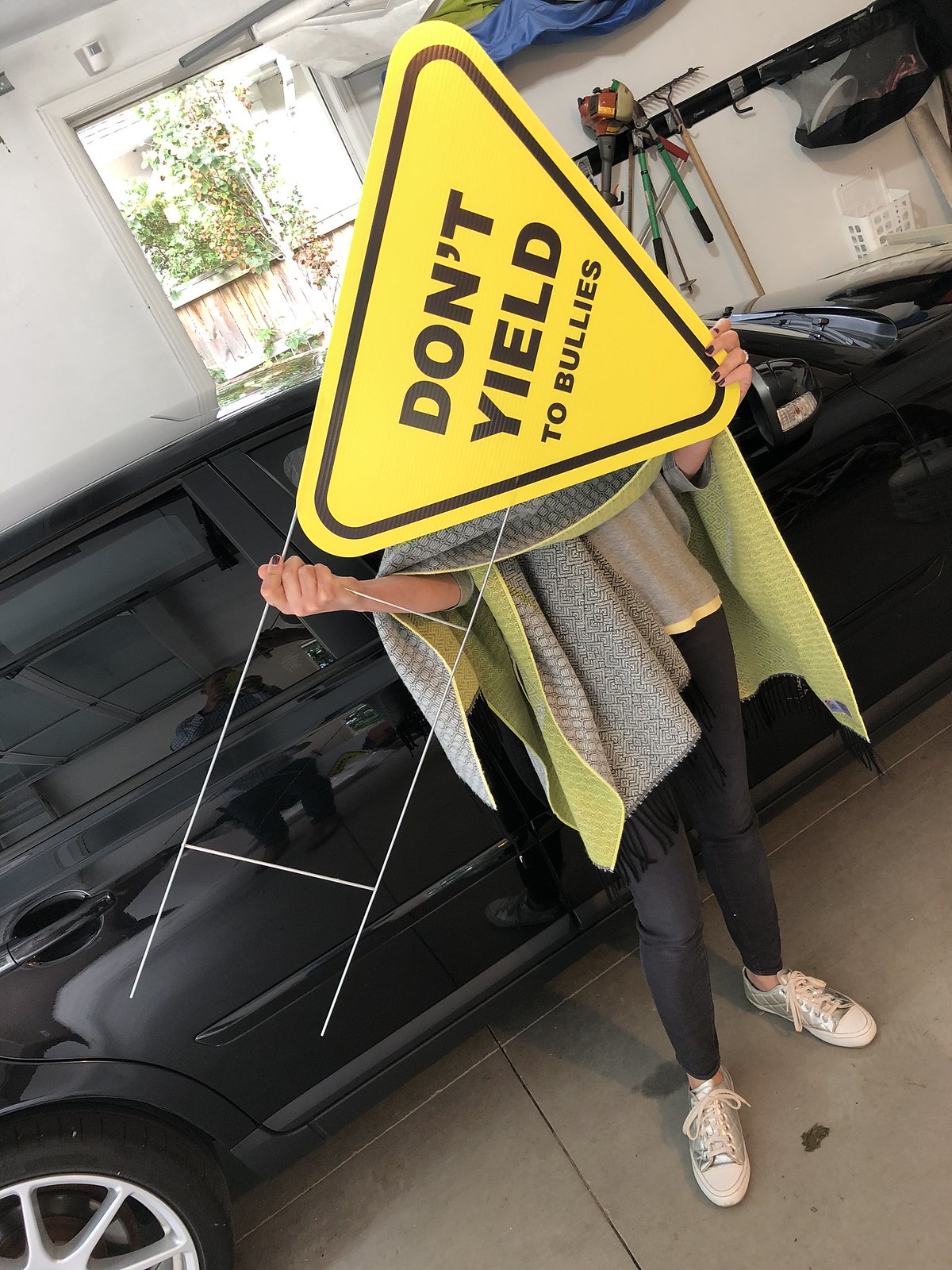This picture features a woman standing in a garage, holding a yellow yield sign outlined in black that says "Don't Yield to Bullies," covering her face. The sign is attached to a thin metal wire base, typically used for yard displays. The garage background includes a white wall with an open doorway in the middle, leading to the side yard with a small tree visible outside. On the right-hand side of the wall, a black hanging rack displays various household tools such as a rake, bolt cutters, trimmers, and a white basket. The woman stands in front of the passenger side of a black two-door car with silver rims. She is dressed in a gray and green poncho over a gray sweatshirt and yellow T-shirt, complemented by black leggings and white-silver tennis shoes with white tips and laces. The floor beneath her is made of concrete.